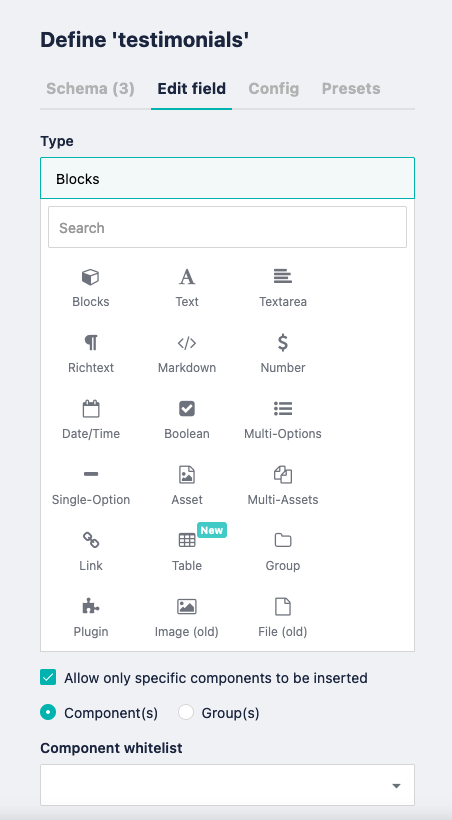This image depicts a web page interface from an unidentified website. At the top left corner, the word "defined" is displayed within quotation marks, followed by "testimonials." The interface offers four clickable options: "Schema (3)," "Edit Field," "Config," and "Presets." 

The screenshot specifically highlights the "Edit Field" section. Below this, there are tabs labeled "Types" and "Blocks," accompanied by a search bar which is currently empty.

A variety of icons and labels are listed under these tabs:
1. **Blocks** - icon of a block.
2. **Text** - icon featuring the letter 'A.'
3. **Text Area** - icon resembling a bar graph.
4. **Rich Text** - icon that is not easily identifiable.
5. **Markdown** - icon of a forward slash.
6. **Number** - icon with a dollar sign.
7. **Date/Time** - icon of a calendar.
8. **Boolean** - icon of a check mark.
9. **Multi Options** - icon with bullet points.
10. **Single Option** - icon with a single line.
11. **Asset** - icon of an image.
12. **Multi Assets** - icon with two image layers.
13. **Links** - icon of a chain link.
14. **Table** - icon of a table grid.
15. **Group** - icon of a folder.
16. **Plugin** - icon of a puzzle piece.
17. **Image** - icon of an image.
18. **File** - icon of a blank piece of paper.